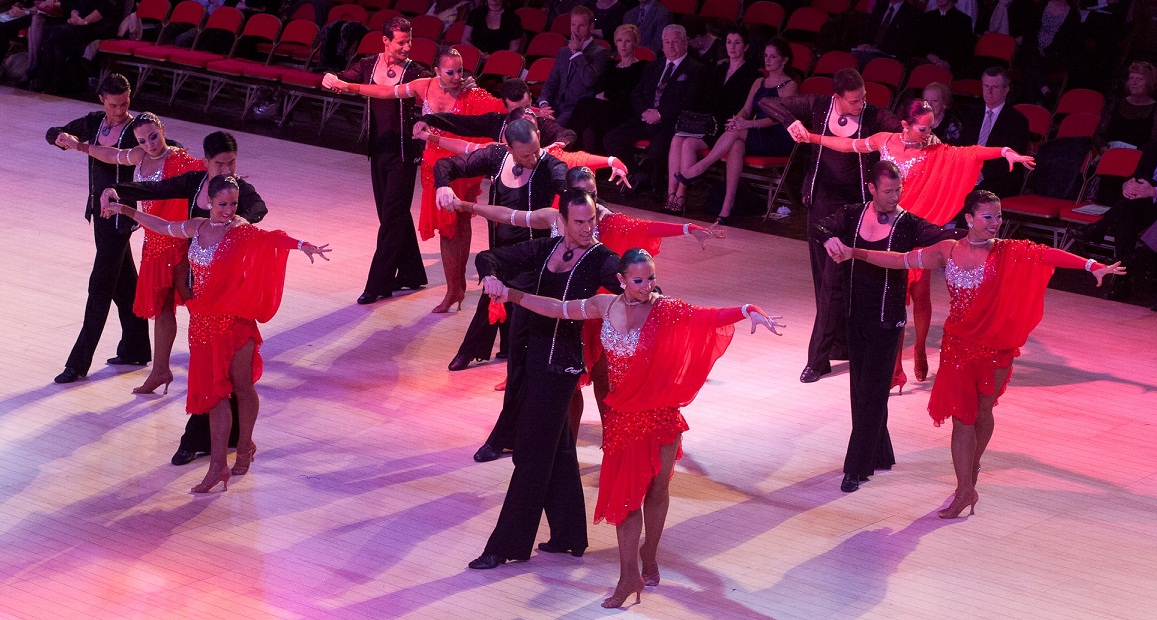The image captures a vibrant performance of samba dancers on a wooden dance floor, suggesting a professional setting such as a theater or dance show. Paired up in a striking ensemble, there are eight couples consisting of one man and one woman each. The women are clad in short, elaborate red dresses with silver embellishments on the bralette area. Their attire is adorned with thoughtful details including left-arm bracelets and right-arm cuffs, complemented by high heels, styled hair, and exquisite makeup. The men are in coordinated black outfits featuring lightweight jackets and matching pants, all accentuated with silver details. The backdrop reveals a large seating area with red chairs where a well-dressed audience in suits and dresses watches intently. The atmosphere suggests a refined, formal event, capturing the audience's anticipation and the dancers' elegant synchronization.